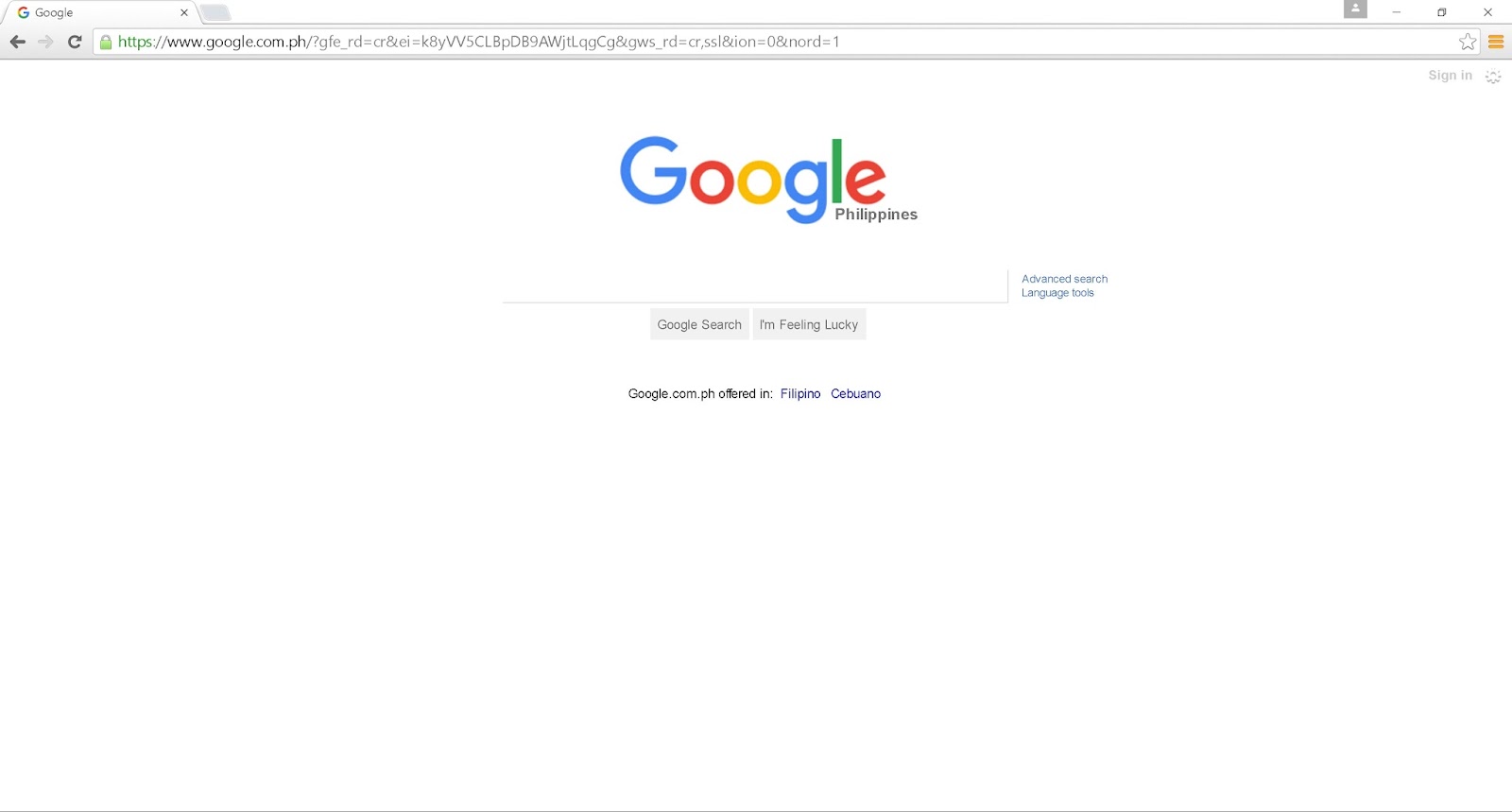A screenshot depicts the Google Philippines homepage set against a white backdrop. The top navigation bar includes a gray left arrow, a lighter gray right arrow, and a refresh button. A star icon and a yellow menu (hamburger) icon are also visible. The screen shows a whimsical illustration featuring a sun and cloud, labeled 'San Ian.' 

Prominently, the Google logo is displayed with its classic multicolors: a blue 'G,' a red 'O,' a yellow 'O,' a blue 'G,' a green 'L,' and a red 'E.' Below it lies the search bar. Below the search bar, in a small font, are links labeled 'Advanced Search' and 'Language.' 

Further down, two gray buttons are visible: one labeled 'Google Search' and the other 'I'm Feeling Lucky.' At the bottom, the text indicates the site is offered in additional languages: 'Filipino' and 'Cebuano.'